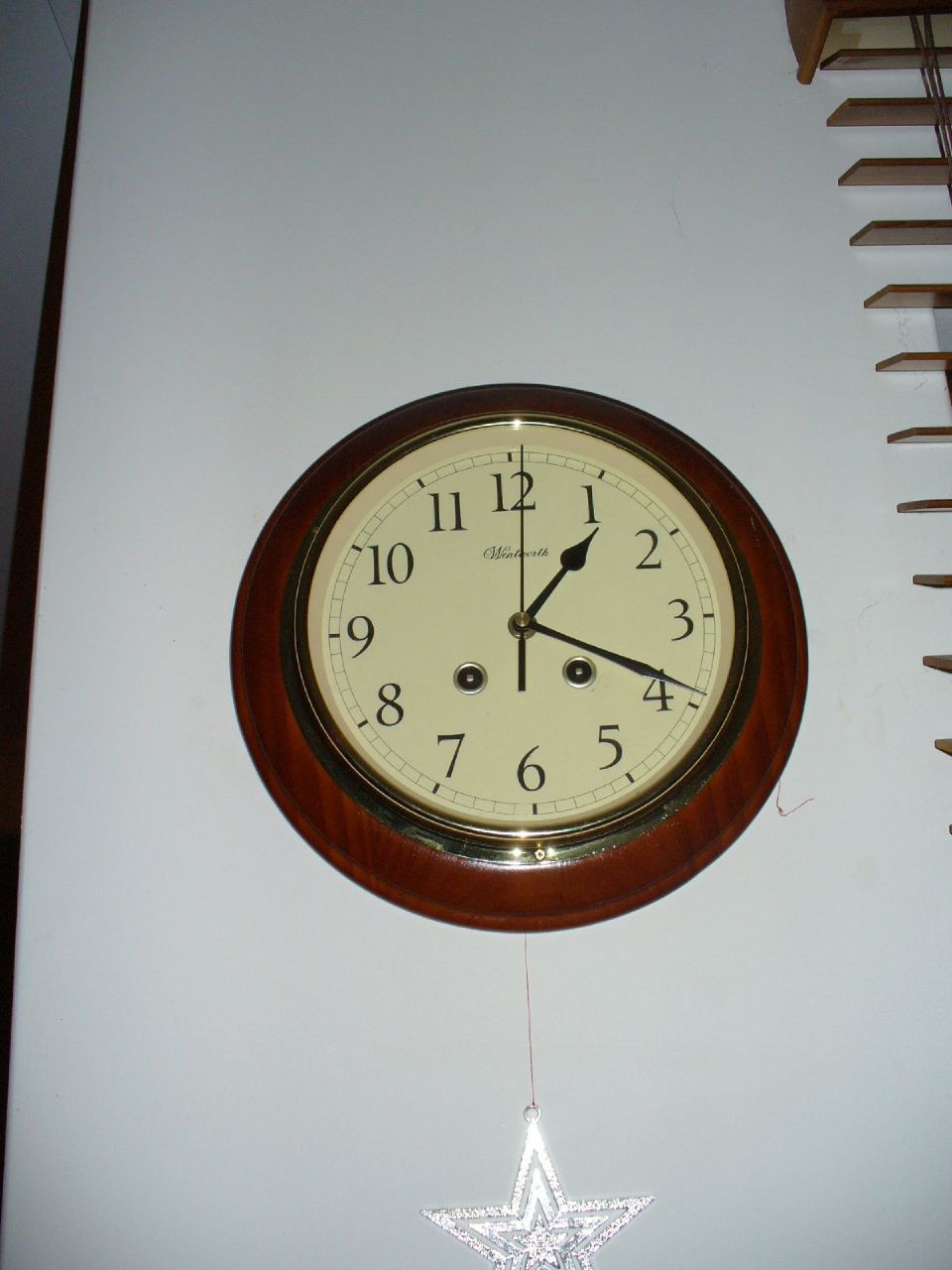The image is of a wall-mounted clock with a wooden outer rim and a plain, vanilla white face adorned with numbers all around it. The minute hand is positioned slightly past 12, the hour hand is a bit past 1, and the middle hand rests just before 4. Notably, there is an insignia beneath the number 12, possibly reading "Williams," indicating the clock brand. The clock is set against a white wall, casting a shadow to the left. To the right, brown wooden or faux wooden blinds are drawn down. A decorative silver star hangs below the clock, adding an extra touch to its appearance.